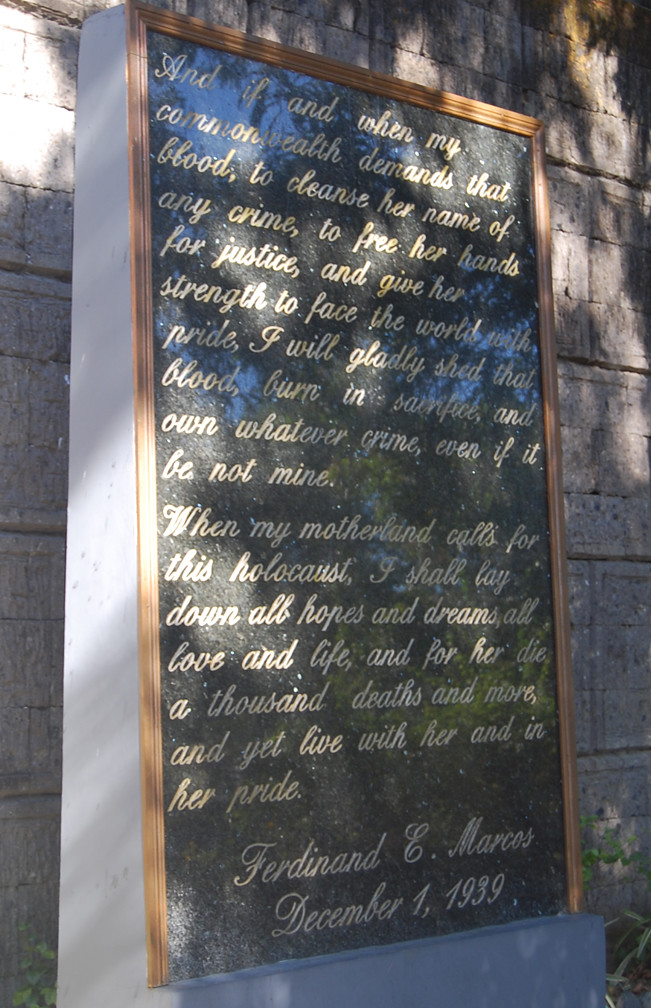The image depicts a solemn outdoor memorial featuring a black stone plaque with a gold frame mounted on a backdrop of gray cinder blocks. The scene is illuminated by sunlight filtering through tree branches casting shadows over the plaque. At the base of the plaque, small shrubs flank either side. The plaque bears an engraved inscription in elegant cursive font, difficult to read from a distance but rich in detail. It eloquently states: "And if and when my Commonwealth demands that blood to cleanse her name of any crime, to free her hands for justice and give her strength to face the world with pride, I will gladly shed that blood, burn in sacrifice, and own whatever crime, even if it be not mine. When my motherland calls for this holocaust, I shall lay down all hopes and dreams, all love and life, and for her die a thousand deaths and more, and yet live with her and in her pride." The quote is followed by the name Ferdinand E. Marcos and the date December 1, 1939.